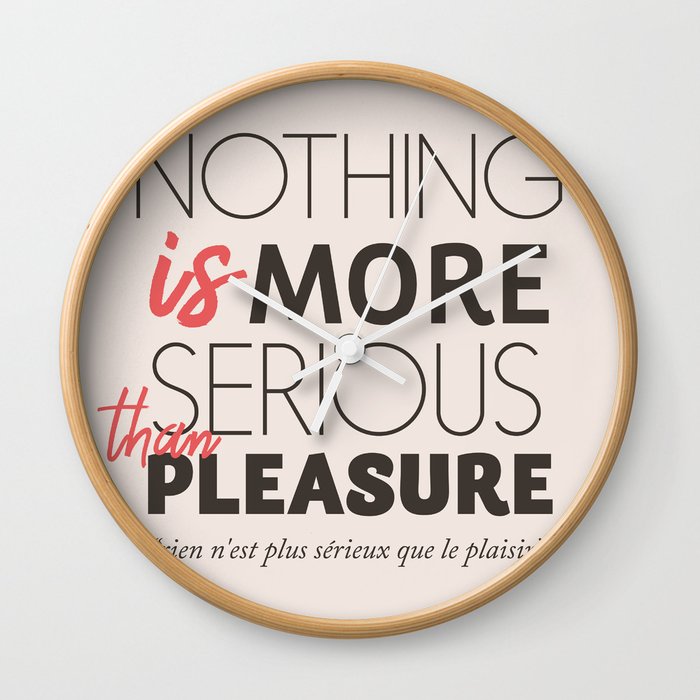The image is a photograph of a round clock featuring a wooden rim set against a white background. The main body of the clock showcases an inscription instead of numbers. Displayed in the center, the phrase "Nothing is more serious than pleasure" is rendered in mixed styles: thin black fonts for 'nothing' and 'serious,' thick black fonts for 'more' and 'pleasure,' and cursive red fonts for 'is' and 'than.' Below this, a smaller French translation appears in standard thin black font. The clock's hands, colored white, include a larger hand pointing towards the top right, another large hand pointing from the left diagonal, and a thin third hand, though they do not indicate an accurate time. The background of the clock is an elegant cream color, and the overall text design emphasizes the playful yet serious message with its contrasting fonts and colors.